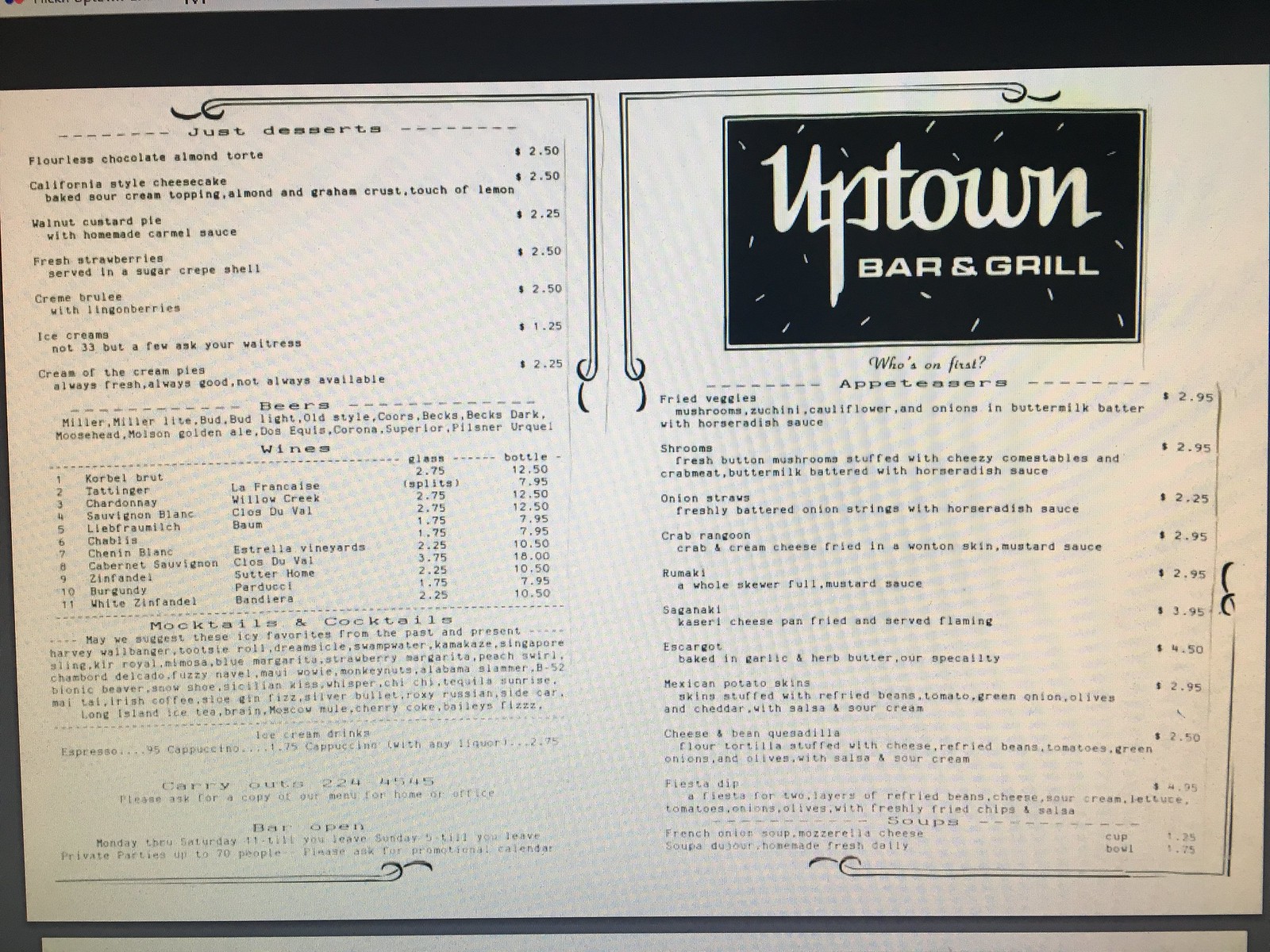The image features a menu from Uptown Bar & Grill. The menu design utilizes a predominantly black and cream color scheme, with "Uptown" in elegant cream-colored lettering and "Bar & Grill" in all capital letters of the same hue against a black background. The content is divided into multiple sections with distinct headings. 

On the right side, there is a category called "Who's on First," listing items such as fried veggies, onion rings, crab dishes, and more. However, the text becomes progressively smaller and lighter towards the bottom, making it challenging to read.

The menu is adorned with an L-shaped decorative border, framing the right corner and the left corner at the bottom. The bottom section on the right side is labeled "Just Desserts," listing various dessert options. The layout is mirrored with another L-shaped pattern on the upper right side, minus the vertical line, which only extends horizontally.

The middle section features an extensive array of beverages, including beers, a lengthy selection of wines, mocktails, and cocktails. Similar to the rest of the menu, the text fades and becomes lighter towards the bottom.

Overall, the menu exudes a sophisticated black and cream aesthetic, resting on a black background. The cream-colored print of "Uptown Bar & Grill" stands out prominently at the top, encapsulating the classy yet contemporary vibe of the establishment.